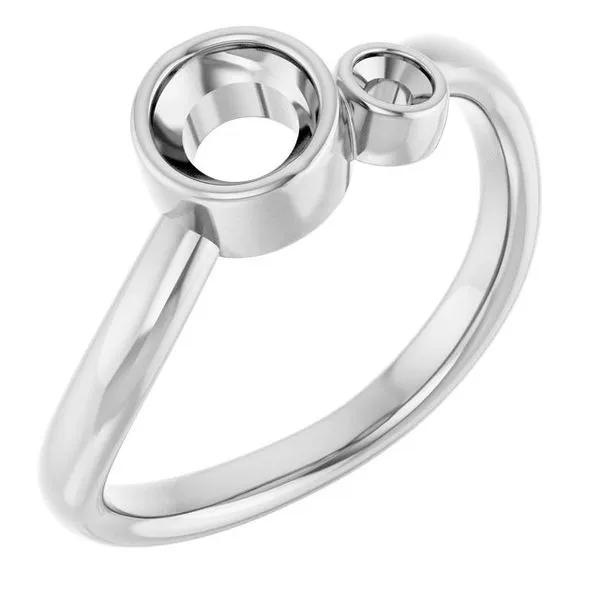This is an intricately designed silver ring, set against a stark white background that accentuates its polished finish. The ring is showcased diagonally, with the broader section pointing towards the lower left of the image. This ring features a D-shaped cross-section, where the outer surface is curved and the inner part, which would rest against the finger, is flat. A notable detail is its seemingly deliberate slight warping towards the left side of the ring. The top part of the ring, presumably the setting area, is hollow and comprises two empty circular cavities — the larger one on the left, likely intended for a primary stone such as a diamond, and a smaller one to its right for an additional gem. The minimalistic and well-lit background, typical of product advertisements, emphasizes the ring's highly polished and pristine condition, free from any noticeable damage or imperfections.